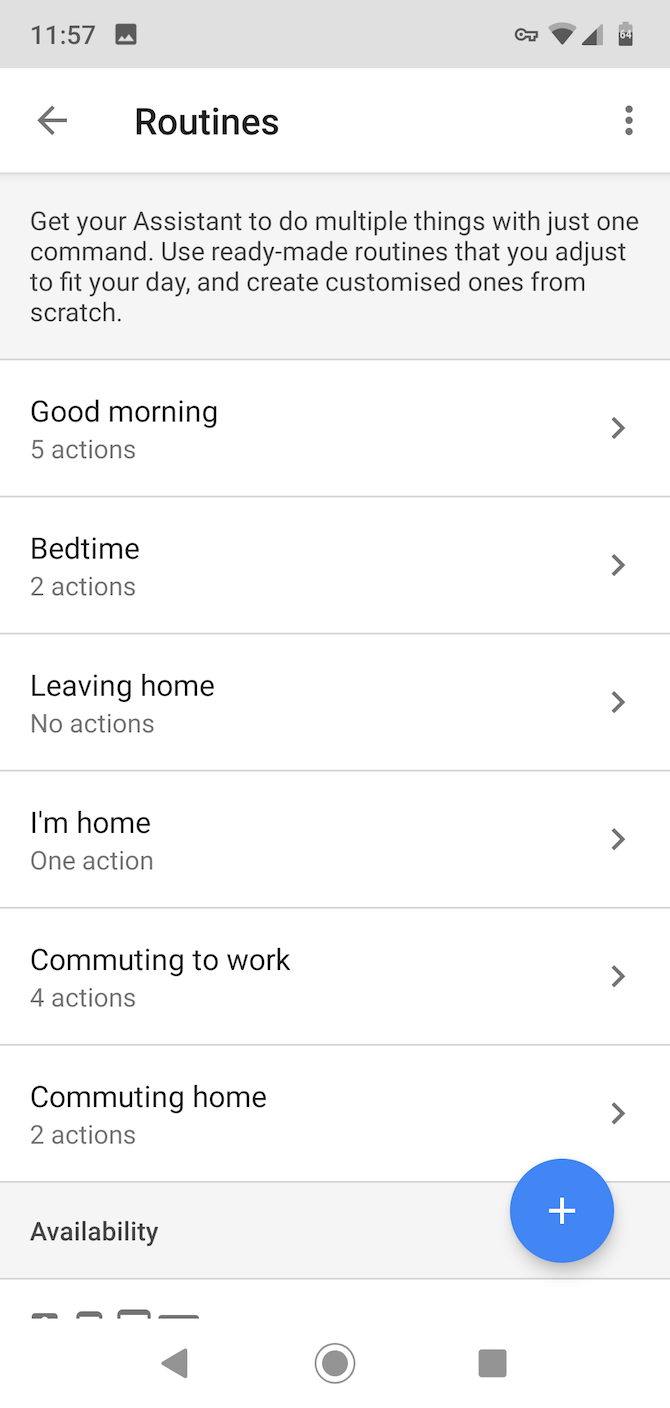This image is a detailed screenshot of the "Routines" settings page on a smartphone, likely for a virtual assistant. The smartphone's status bar is visible at the top; it displays the time as 11:57 AM on the left and indicates that the battery is approximately 25% charged on the right. 

The "Routines" section at the top of the page is designed for configuring the assistant's behavior in response to specific commands or triggers. The header explains that users can enable their assistant to perform multiple actions with a single command, featuring both pre-made routines that can be customized and options to create new routines from scratch.

Listed below the header are several default routines:
- **Good Morning:** Activates five actions when the command is issued.
- **Bedtime:** Activates two actions.
- **Leaving Home:** Currently has no actions assigned.
- **I'm Home:** Triggers one action.
- **Commuting to Work:** Initiates four actions.
- **Commuting Home:** Initiates two actions.

At the bottom of the screenshot, the "Availability" section indicates where the user can manage the accessibility of these routines.